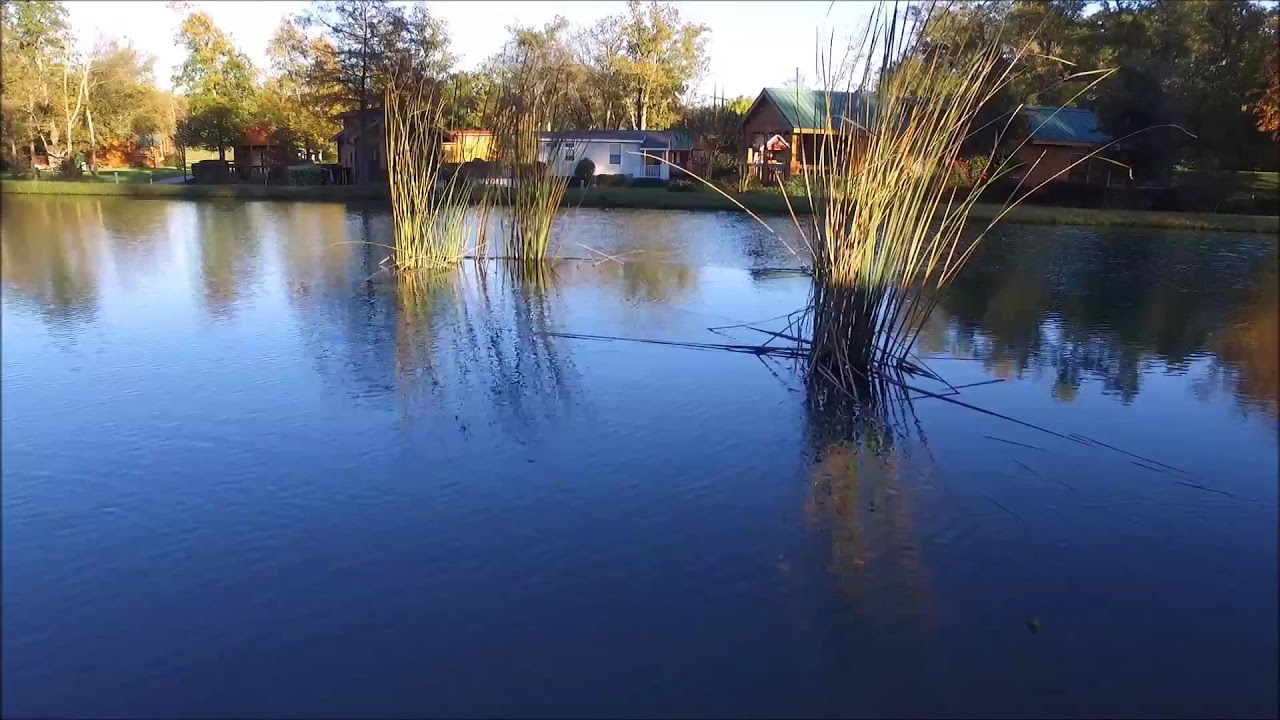This image depicts a serene lakeside scene on a clear, bright day. Dominating the foreground is a calm lake, occupying about two-thirds of the image, with its smooth surface reflecting the surrounding scenery. Scattered within the lake are clusters of tall reeds or seagrass, positioned toward the center and right side of the water. Along the shoreline, lush green grass extends up to a row of picturesque lake houses. These houses vary in appearance, including a charming log cabin with a green metal triangular roof and a white single-story house with black tiled roofing. Behind the houses, dense trees, their leaves beginning to change color, hint at the onset of fall. There is no text in the image, and no people are visible, accentuating the peacefulness of the scene. The colors are vibrant, with blues of the water, greens of the reeds and trees, and a mix of whites, browns, and greens from the houses, collectively creating a tranquil and inviting landscape.